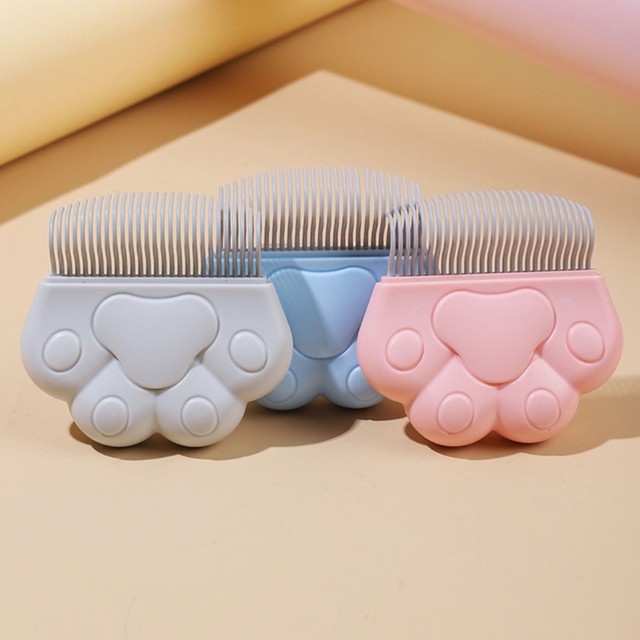The image is a detailed color photograph, possibly computer-generated, showcasing three plastic objects that resemble combs or grooming tools. Each object is shaped like a pet's paw, complete with etchings of four smaller pads and a larger central pad. The objects are positioned upright on a light pink surface. The object on the left is light gray, the one in the center is light blue, and the one on the right is light pink. Above the plastic paw-like bases are rows of metal prongs, approximately 20 on each object, slightly curving outwards, presumably designed for scraping fleas or flea dirt from animal fur. The light source appears to come from the left, casting shadows to the right.